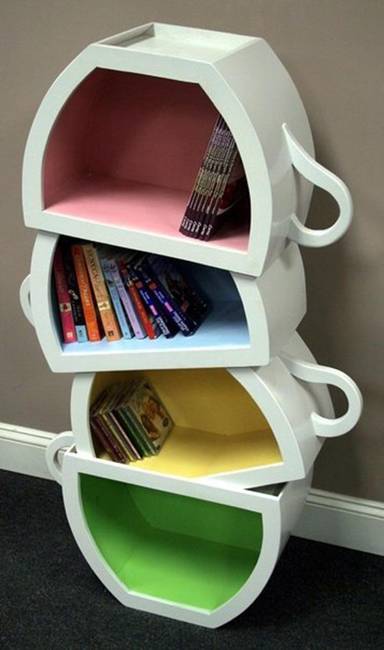This photograph depicts an extraordinary bookshelf designed to resemble four stacked teacups. Each teacup shelf is cut in half, with the top three teacups upturned and the bottom one set upright, creating a whimsical, haphazard stack that leans slightly rather than aligning in a straight column. The inside of each teacup is painted a different color: the top teacup is pink, followed by a blue one, then a yellow one, and finally, at the bottom, a green teacup. The exterior of all the teacups is white. The top shelf holds some magazines, the second blue shelf contains a variety of books, the third yellow shelf has a collection of CDs, and the bottom green shelf is currently empty. This creative bookshelf is set against a dark gray-brown wall adorned with white trim, and it rests on a dark, carpeted floor.